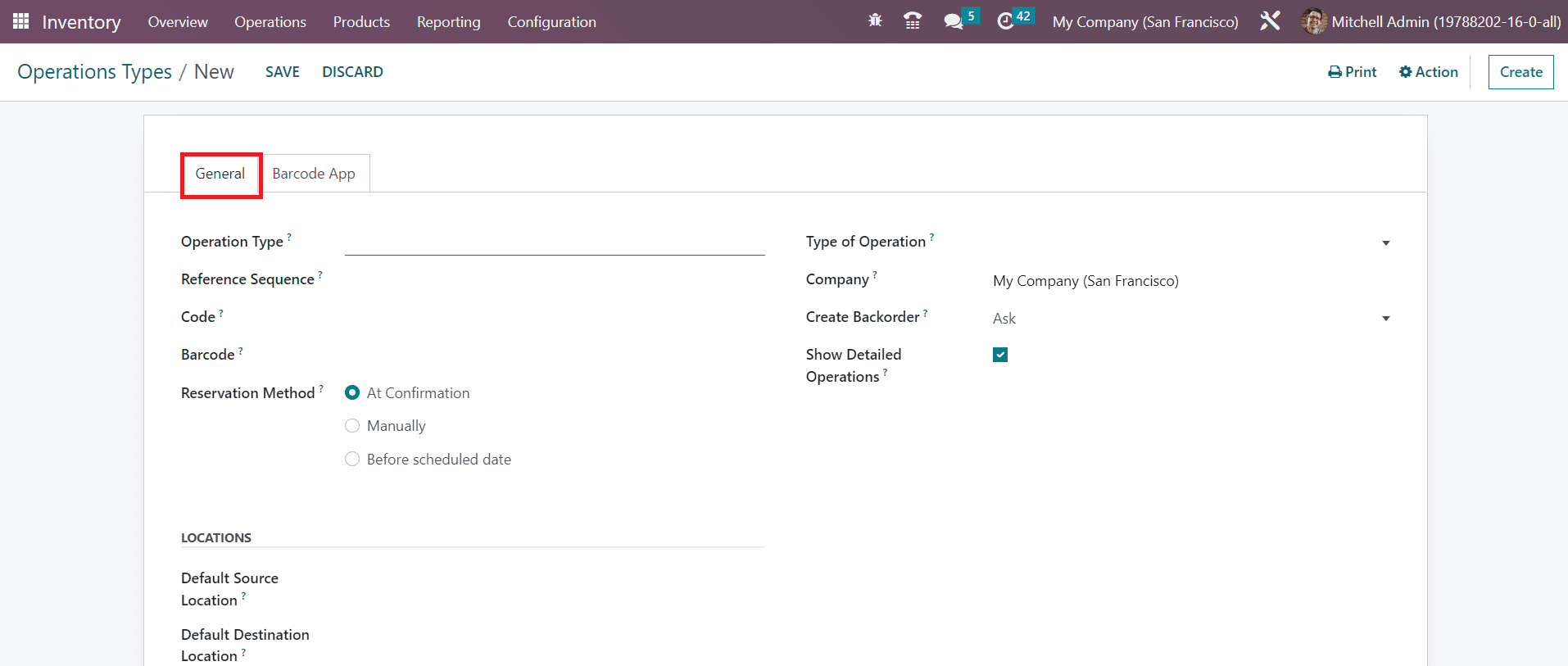This image appears to be a screenshot of a barcode management application, potentially used within a company’s inventory or operation system. The top navigation bar features a purple background and includes various sections labeled: Inventory, Overview, Operations, Products, Reporting, and Configuration, indicating a comprehensive suite of tools for managing different aspects of the business. On the top right corner, the user is identified as “Mitchell Admin,” suggesting administrative access to the system.

Just below the main navigation bar, there are several operational commands including New, Save, Discard, Print, Action, and Create, with Print, Action, and Create displayed as interactive buttons.

The main content area of the page is subdivided into two tabs: General and Barcode App. The General tab is highlighted, bordered by a red outline to indicate it is the active view. Within the General tab, several data fields and options are visible, including:

- **Operation Type**
- **Reference Sequence Code**
- **Barcode**
- **Reservation Method:** With selectable options such as At Confirmation, Manually, or Before Scheduled Date.
- **Locations:** Including Default Source Location and Default Destinations Location.
- **Type of Operation**
- **Company**
- **Create Backorder**
- **Show Detailed Operations**

Under these settings, there is additional information indicating this operation pertains to "My Company" based in San Francisco.

The overall presentation suggests a structured and user-configurable environment for managing inventory and operations, albeit the specific functionalities are not entirely clear from the screenshot alone.